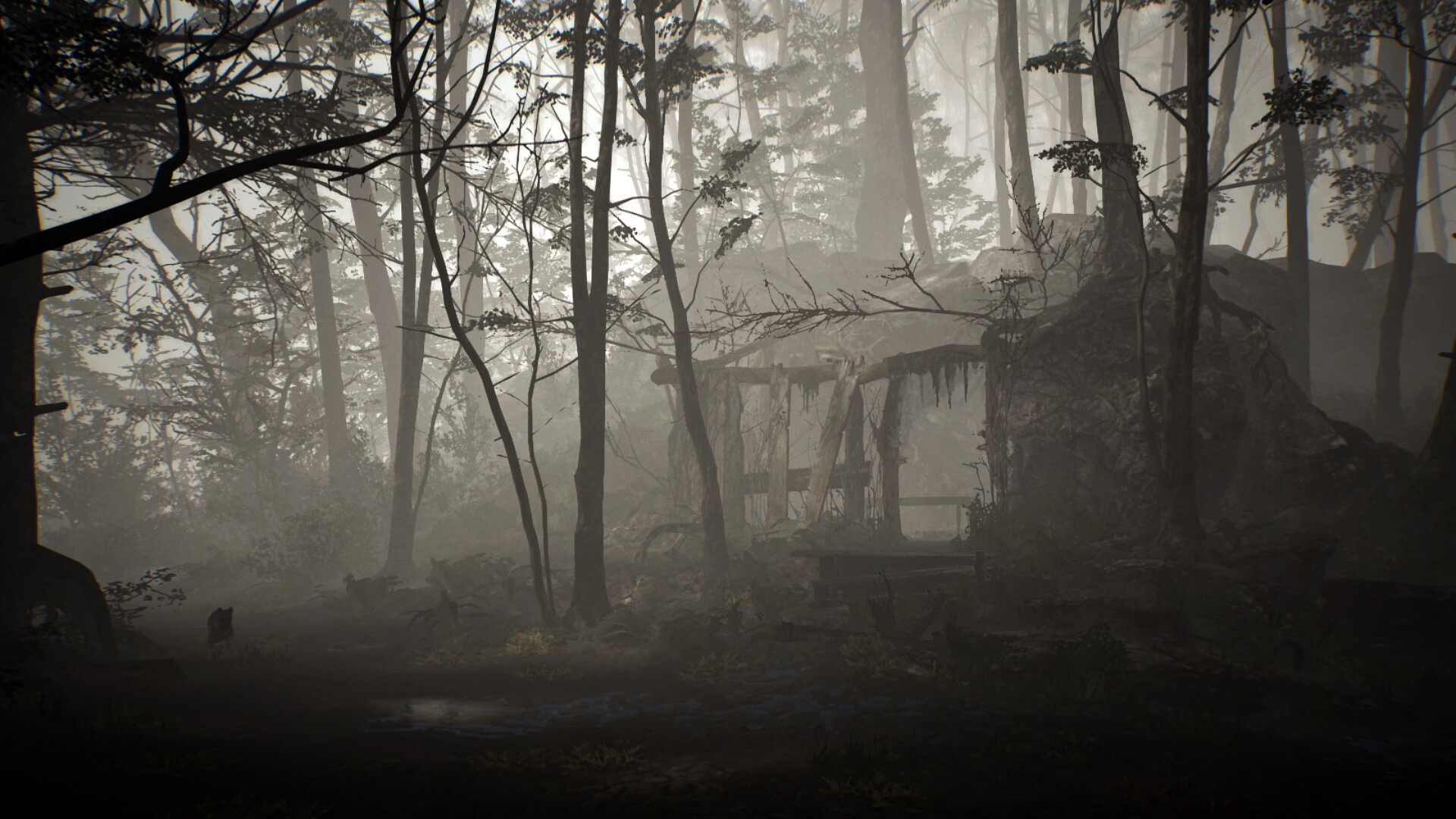This photograph captures a serene, foggy morning within a dense forest. The scene is enveloped in mist, with tall, thin-trunked trees sparsely adorned with leaves, stretching high into the sky. The forest floor is lush and green, with moisture glistening on the foliage, suggesting the freshness of early dawn. To the left of the image, nestled next to a tree, is a small animal, adding a touch of life to the tranquil setting. In the background stands a dilapidated structure, likely an abandoned cabin. Its roof and a few support beams are still intact, but the walls have collapsed, leaving the interior exposed and barren, a testament to its long-forgotten dwellers. Above, the sky is a luminous white, diffused by the fog, creating an ethereal glow that enhances the mystical atmosphere of the forest.